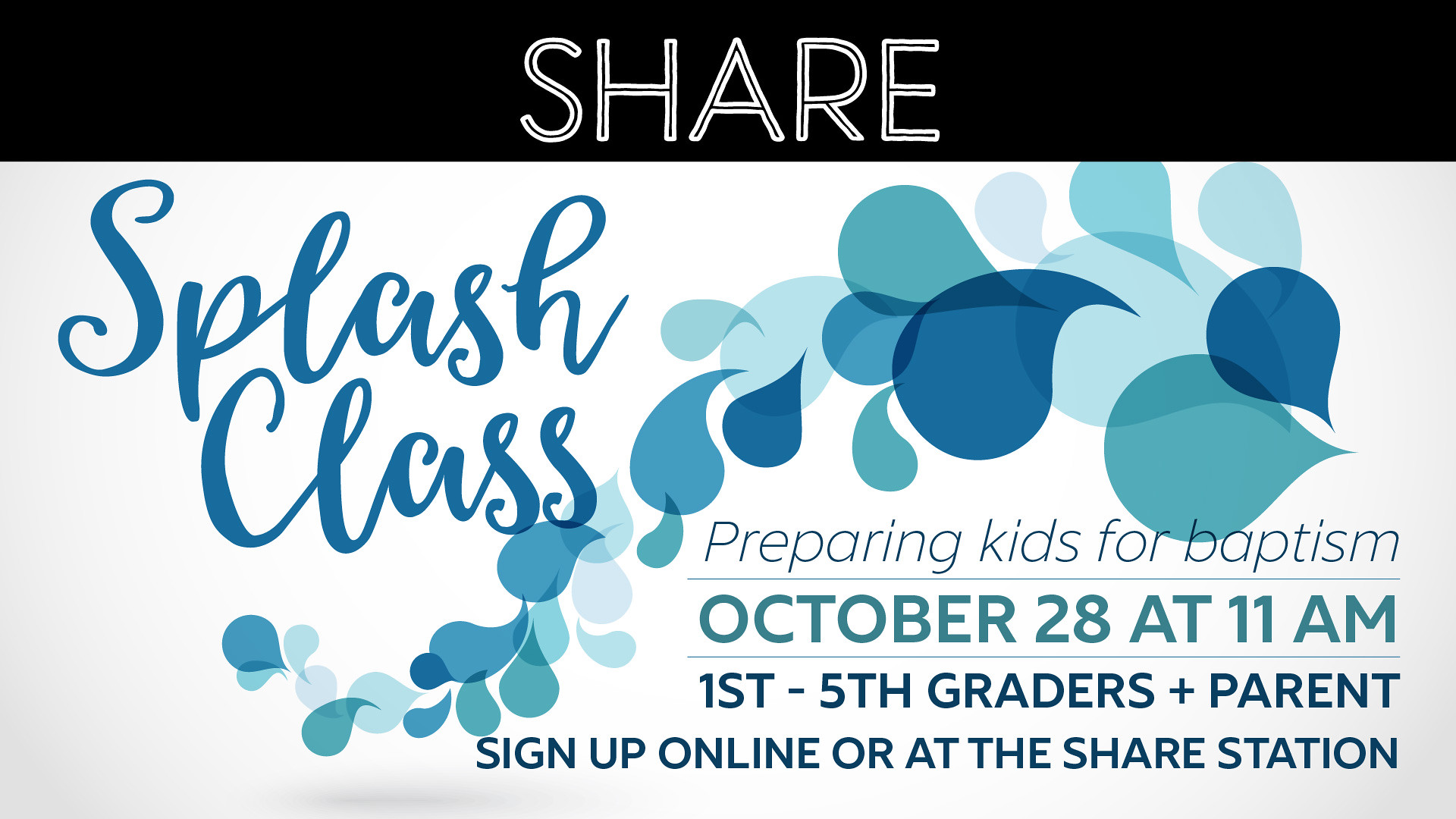**Promotional Banner Description:**

The promotional banner is a rectangular shape with dimensions wider than it is tall, reminiscent of a high-definition TV screen. The very top of the banner features a black strip with bold, white-bordered text in all caps that reads "SHARE." Below the black banner, the rest of the background is light gray. Positioned in the top left section, there is blue cursive text that reads "Splash Class." Stylized blue water drops of varying sizes and shades flow through the center of the image. In the bottom right, black block text announces "Preparing Kids for Baptism" followed by details: "October 28th at 11am," and further instructions, "First to fifth graders plus parent sign up online or at the SHARE station."